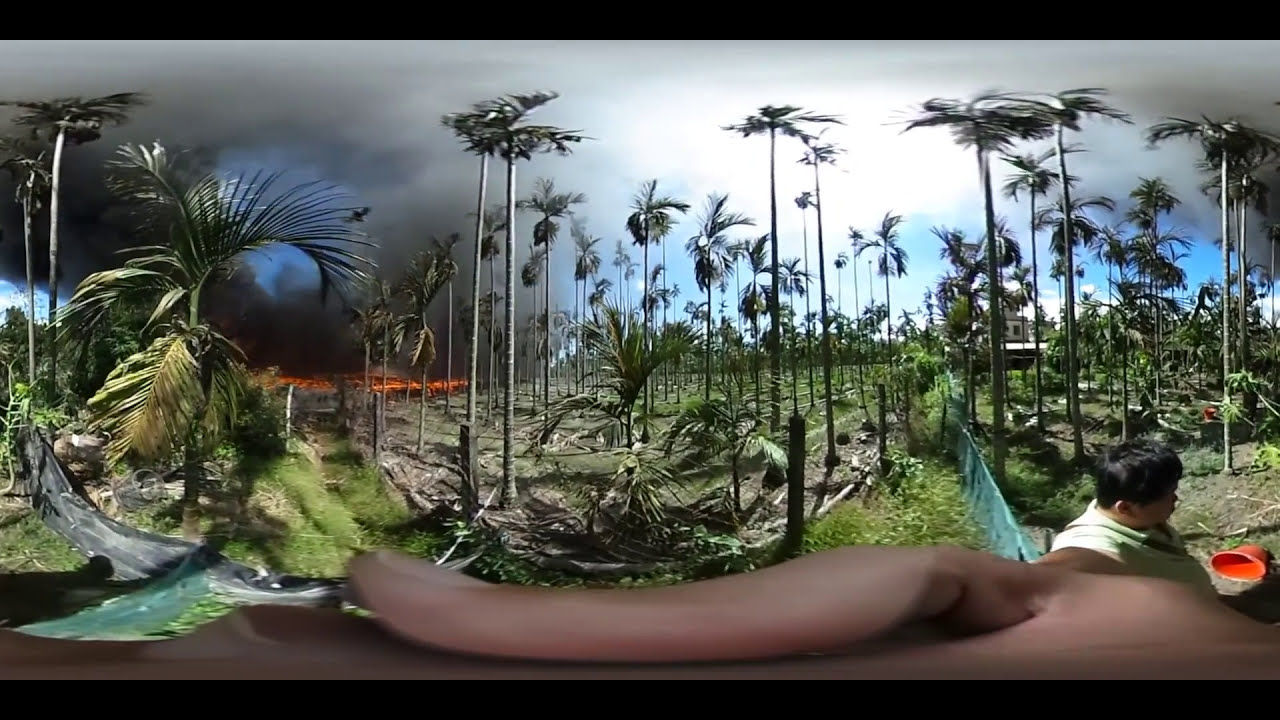In this detailed and bustling scene, we have a slightly distorted color photograph capturing the vibrant, yet somewhat muted elements of a farm or field. Dominating the lower part of the image is a person's hand with a light brown finger positioned prominently at the bottom, suggesting they are taking a selfie. This individual, wearing a light green shirt and black hair, is placed in the bottom right corner.

Surrounding them in the background are fields filled with dozens of tall, swaying palm trees, indicating a windy day. Interspersed among these trees are various farm structures, including a house in the middle right section and numerous black and light blue fencing segments. To the left of center, a burning field spews black and gray smoke into the sky, hinting at a controlled burn. This smoky chaos contrasts with patches of serene, clear blue sky and white clouds, to the right of the image.

Nearby, an orange bucket lies tipped over on the ground, suggestive of recent activity. The grassy landscape is dotted with black and green barriers, perhaps demarcating areas within the farm. Altogether, this vivid image captures a moment rich with natural and human elements, portraying a day filled with activity and swirling weather patterns.